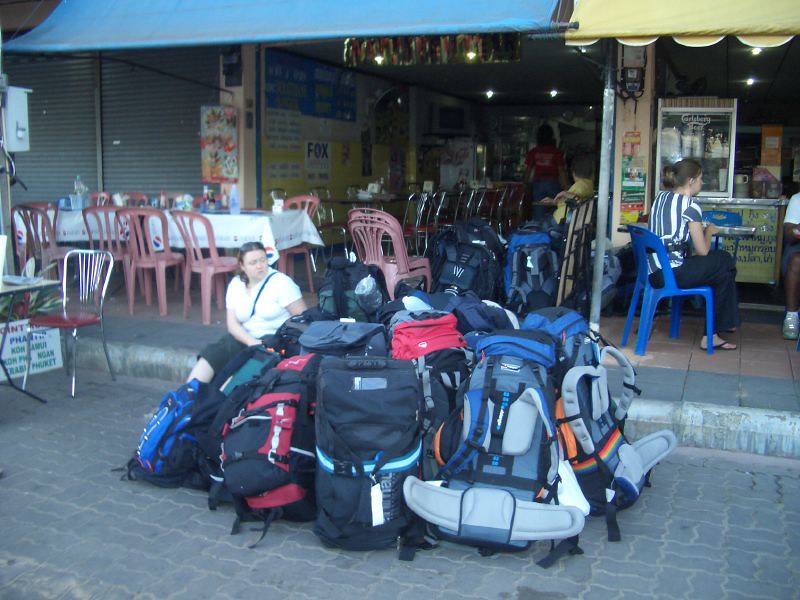This outdoor photograph captures a well-maintained, cobblestone street with irregular-shaped stones and a clean, though slightly dirty, concrete curb. Central to the image is a closely packed pile of about 9 or 10 colorful backpacks—some blue, black, and red—each designed for carrying on one's back and appearing full, possibly awaiting transport. Flanking this pile, a woman with brown hair, dressed in a white t-shirt and black shorts with a ribbon, sits on the curb looking off-frame with a purse on her shoulder.

In the background, there is an open-air restaurant with many wooden tables and chairs, some shaded by a blue cover and a yellow shutter. The restaurant is dimly lit, and a person in a red shirt with white writing is seen walking through. Adjacent to the restaurant is a food stand with a glass box containing disposable cups and dishes. In front of this food stand, another woman, seated on a blue chair at a small table, is wearing a white and black t-shirt and black pants, with her brown hair tied in a ponytail. Other people are faintly visible in the background, sitting outside the restaurant, creating a lively but relaxed atmosphere.